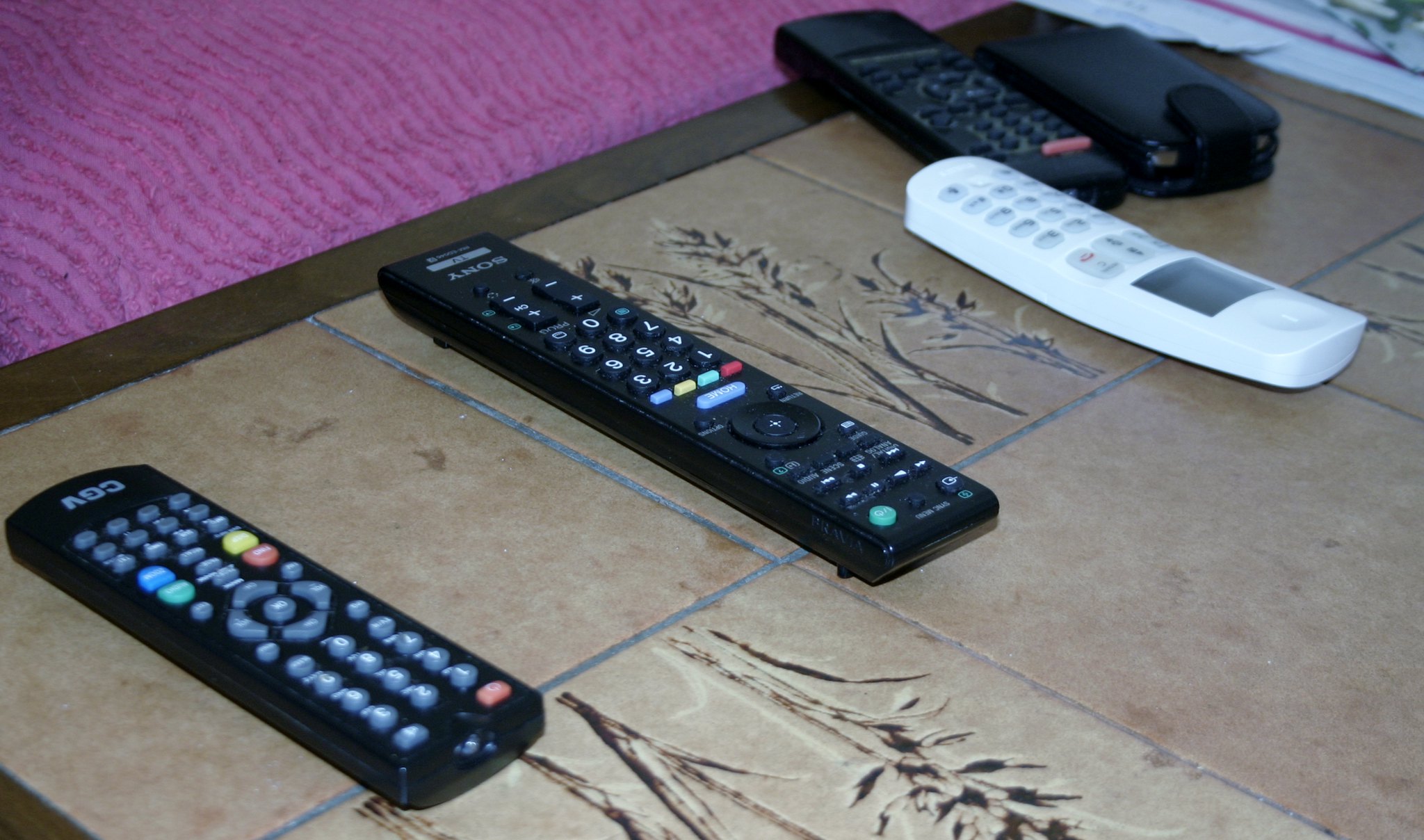The image displays an array of remote controls scattered on a tiled floor. The floor tiles, which are light brown, feature engravings of plants and flowers on some of the squares, while others remain plain. The scene is framed by a wooden border around the tiles, suggesting the surface could be either a table or a sectioned-off floor area. A textured pink carpet with darker pink wavy lines appears along the left edge of the image.

Centrally placed among the remotes is a white wireless phone with opaque buttons, a small LCD screen, and a hang-up symbol. To the left of the phone, a remote labeled "CGV" with a distinct red power button stands out. Next to it, another remote marked "Sony TV" features a green power button. Positioned at the farthest left is a somewhat indistinct black remote with a prominent red button.

On the right side of the phone, there is a black object resembling a phone case, potentially holding a phone. Another black remote with a pink pattern lies adjacent to a black wallet on the top right of the image. This assortment of devices suggests the area is close to an entertainment setup, given the diversity and number of remotes.